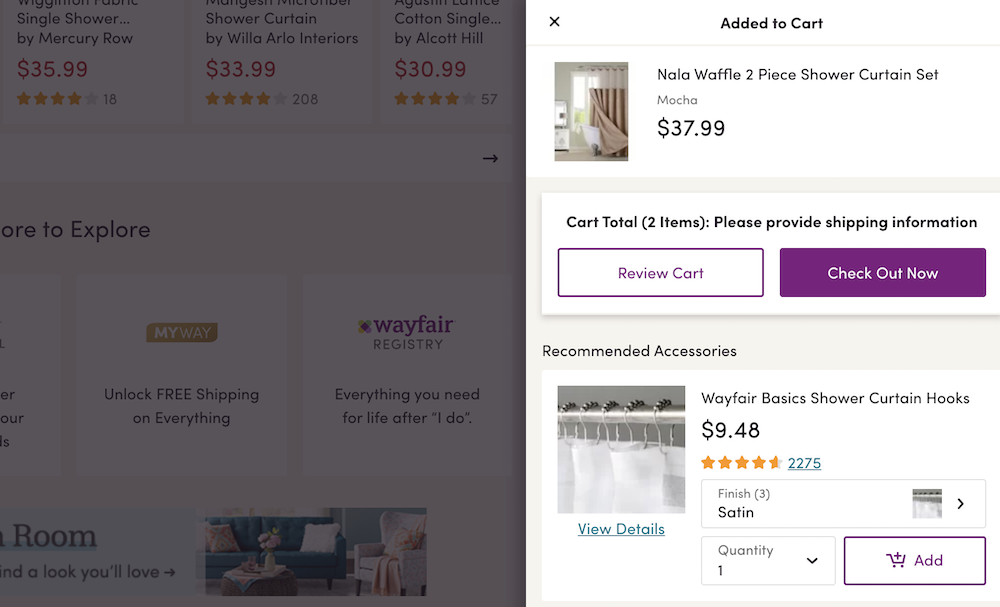This image depicts a shopping experience, either on a cell phone or a computer. The left side of the screen is dimmed with a gray overlay, drawing attention to the right side where the cart information is displayed prominently. On the left, albeit less visible, there are several elements including a "My Way" section for unlocking free shipping, a Wayfair registry promoting everything needed for post-wedding life, and partially visible ratings and prices for various items. Notably mentioned are a single shower curtain made of cotton.

On the right side, the cart interface is highlighted. At the top, it shows that a "Nala Waffle Two-Piece Shower Curtain Set" in Matcha color has been added to the cart, priced at $37.99. The cart currently contains two items, and the user is prompted to provide shipping information. Two prominent buttons allow the user to either "Review Cart" or "Checkout Now," with the former in white and the latter in purple. At the bottom, there is a "Recommended Accessories" section featuring shower curtain hooks.